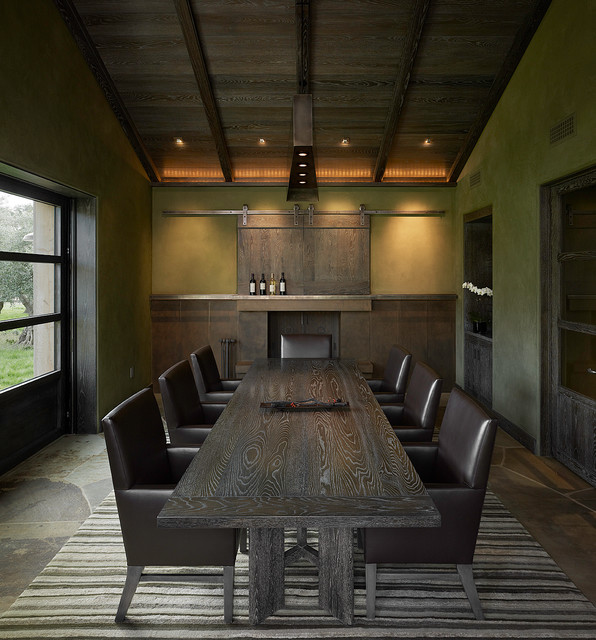The image depicts a dark, masculine boardroom or tasting room with an inviting, cozy ambiance. A long, dark wood table stretches down the center of the room, featuring a unique U-shaped leg design. Surrounding the table are seven square-shaped, solid brown leather chairs, each with matching wooden legs and armrests. The table rests on a brown and white striped carpet that adds texture to the wooden floor beneath.

The room is enveloped in various shades of green, with the left and back walls painted a deep green, and the right wall featuring two doors. A stone fireplace adorned with a wooden mantel stands at the far end of the room, holding four bottles of what appears to be wine. Above, wooden beams grace the ceiling, which houses four lights that softly illuminate the space. A shelving unit in the back adds a touch of rustic charm, while large windows resembling a converted garage door on one side allow natural, rainy light to seep in, contrasting with the room's dark, cozy atmosphere. Despite its moody tones, the space feels welcoming and is perfectly suited for intimate discussions or leisurely tastings.